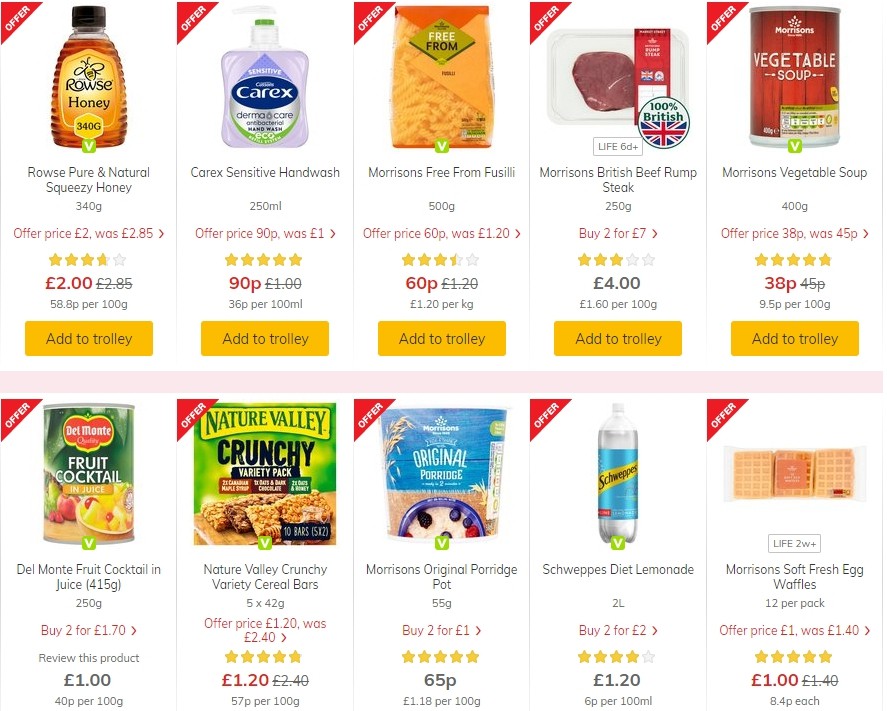This is a screenshot capturing an online shopping interface primarily featuring affordable groceries. The layout consists of two horizontal rows, each containing five items. The top row includes the following products: Carex Dermacare, Fusilli Pasta, British Beef Rump Steak, and Morrison's Vegetable Soup. The bottom row showcases Del Monte Fruit Cocktail, Nature Valley Crunchy Variety Pack cereal bars, Morrison's Original Porridge Pot, Schweppes Diet Lemonade, and Morrison's Soft Fresh Egg Waffles. 

Each item's price is listed in British Pounds, with visible discounts highlighted in red text indicating the original price and the current offer price. Additionally, all ten items are marked with “offer,” signaling special deals. The interface provides an "add to trolley" button beneath the product listings in the top row, facilitating easy addition to the virtual shopping cart. 

Weights of the items are displayed in metric units. A subtle pink line horizontally separates the two rows, and vertical gray lines discretely partition each item. The background is a clean white, ensuring product images and details are clearly visible.